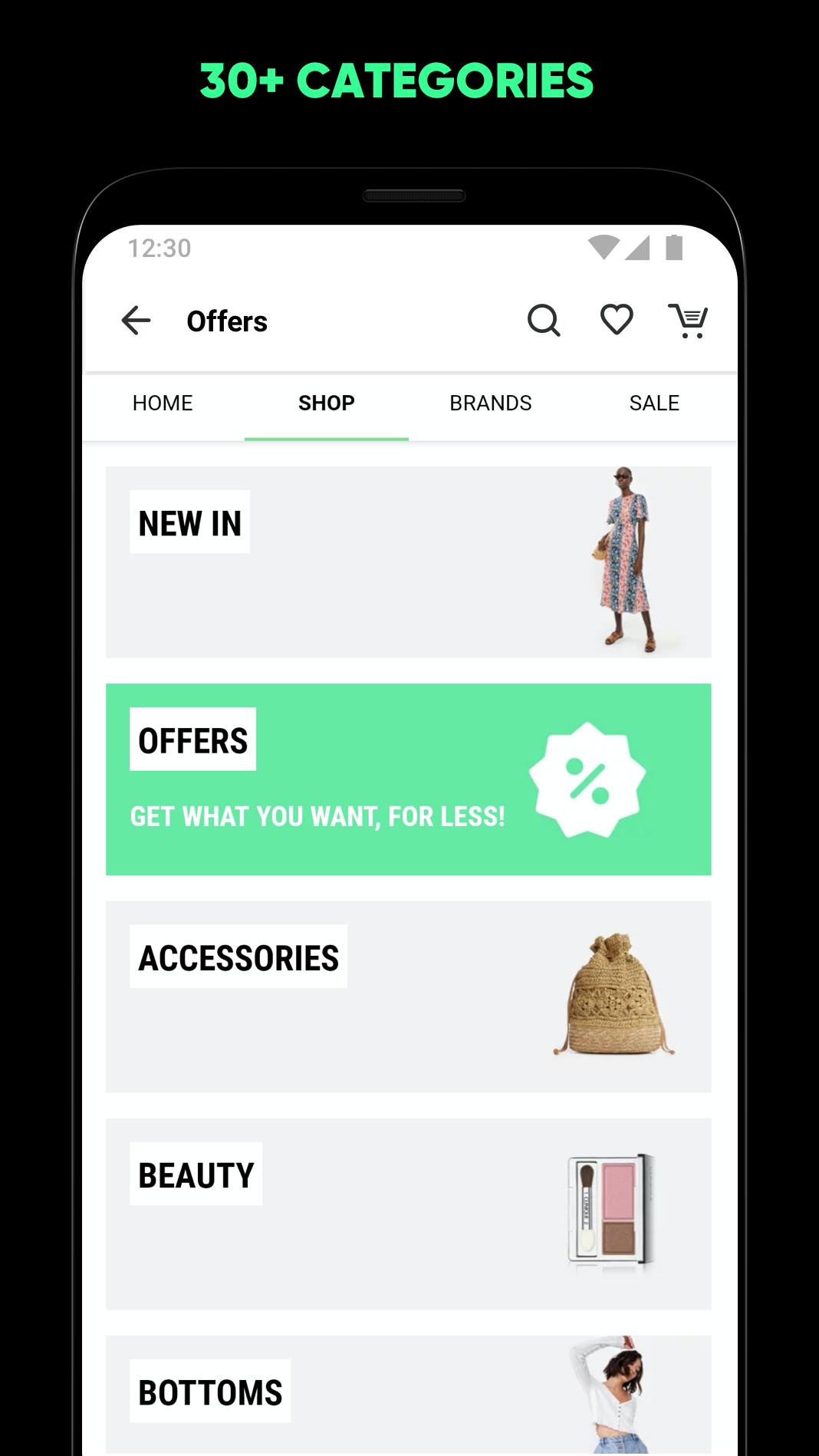The image portrays a web page displayed on a cell phone, characterized by its elongated vertical rectangle shape with a distinct black border on the top section and along the left and right edges. At the top of this black-bordered section, bold green capital letters prominently display the phrase "30+ CATEGORIES." Centered within the black border, a white background features the time "12:30" written in gray letters at the top, accompanied by three icons on the right side: a battery indicator, a wireless signal strength icon, and below them, a partial web page.

The partial web page displays the word "OFFERS" next to a magnifying glass icon, followed by a heart icon and a shopping cart icon in sequence to its right. Below this header, there are navigation categories presented in black capital letters: "HOME," "SHOP," "BRANDS," and "SELL." The "SHOP" section is currently active, as evidenced by its highlighted state.

Underneath the active "SHOP" section, several categories are listed on the left side, each in black capital letters: "NEW IN," "OFFERS," "ACCESSORIES," "BEAUTY," and "BOTTOMS." Corresponding to these categories, on the right side, are small thumbnail images that provide visual representations of what each category entails.